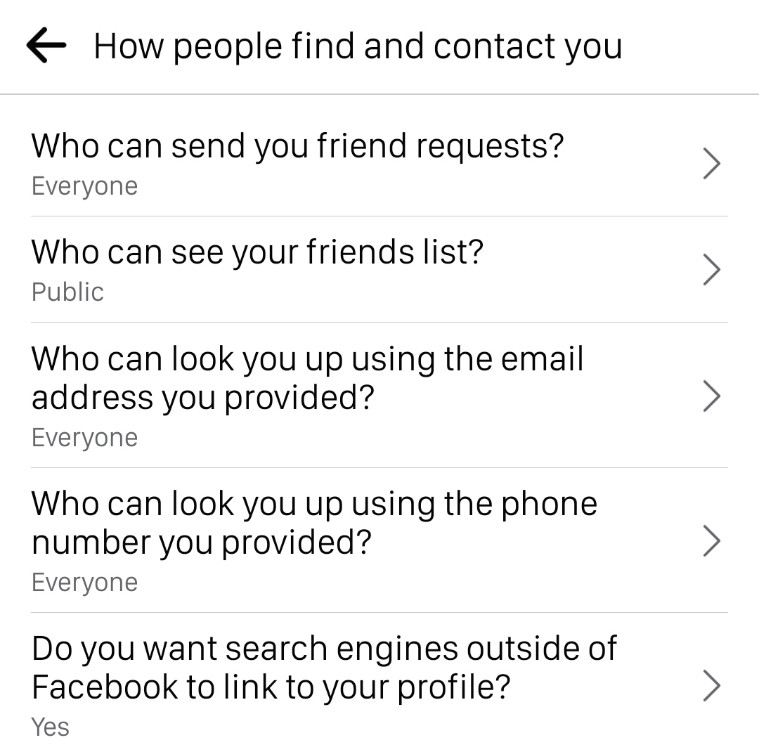The image depicts a section of a large screen showing a privacy settings interface, likely from a social media platform. At the very top, a bolded left-pointing arrow is visible, accompanied by black text that reads, "How people find and contact you." Directly below this is a fine grey line separating the header from subsequent settings.

The first heading, titled "Who can send you friend requests," is currently configured to "Everyone." It is displayed in light grey with a small right-pointing arrow indicating it can be expanded or reconfigured. The second heading, "Who can see your friends list," is set to "Public" and also features an adjustable setting.

Following this, the third heading states, "Who can look you up using the email address you provided." This is set to "Everyone" and is adjustable as well. Similarly, the fourth heading, "Who can look you up using the phone number you provided," is configured to "Everyone," with the option to change it.

Finally, there is a setting, "Do you want search engines outside of Facebook to link to your profile?" currently set to "Yes." Each of these five settings includes a small right-pointing arrow on the right-hand side, indicating that they can be clicked to reconfigure to different values if desired.